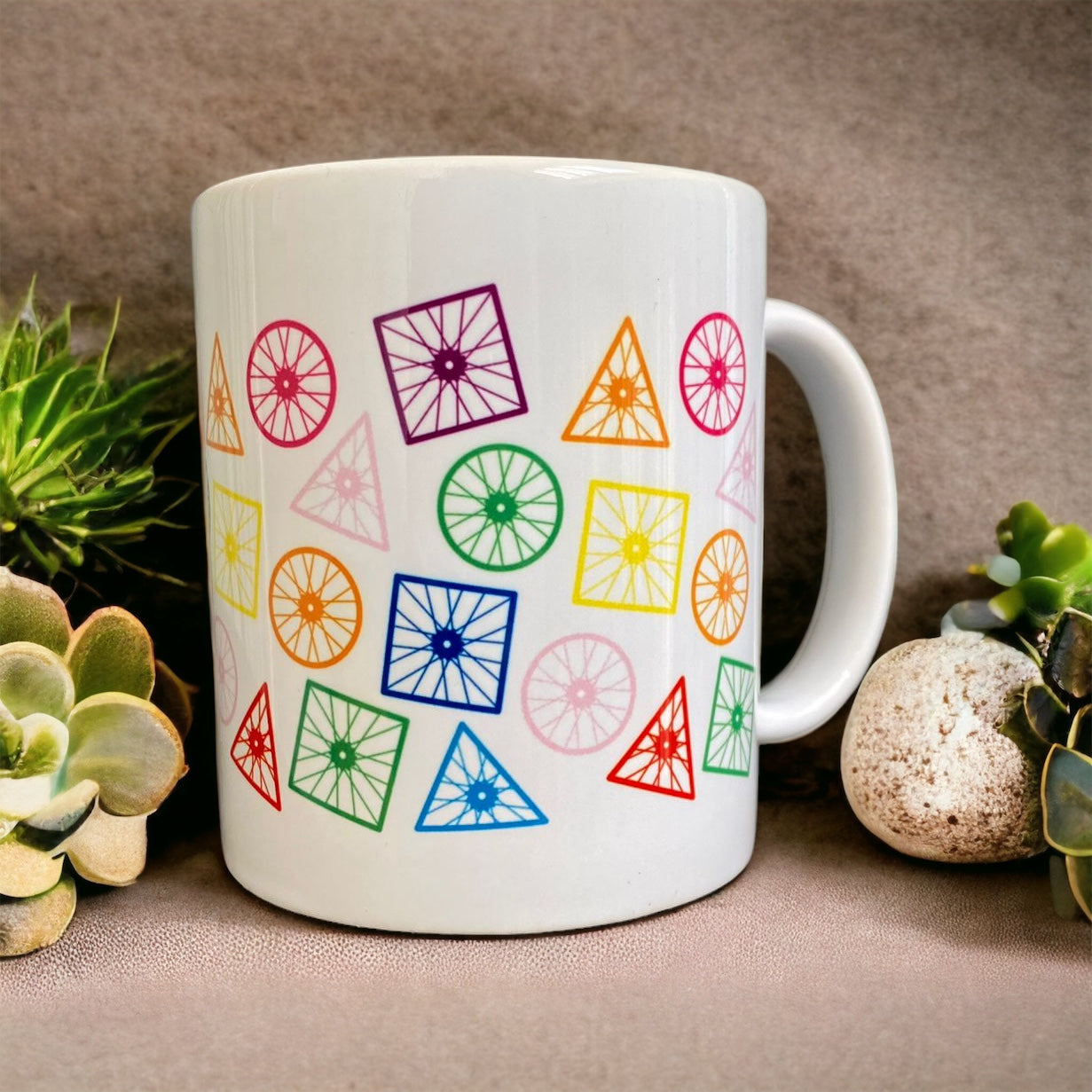This image presents a detailed view of a white ceramic coffee cup adorned with a lively pattern of multi-colored geometric shapes, reminiscent of bicycle wheels. The designs include circles, squares, and triangles, each featuring a solid color at the center and radiating lines or spokes extending outward. The palette spans a spectrum of vibrant hues, including pink, yellow, orange, blue, green, red, and purple.

The cup's handle is prominently displayed on the right, indicating a traditional orientation. It rests upon a tan surface that some interpretations suggest could be an upholstered cushion. To the left of the cup, succulent plants add a touch of natural greenery, while a stone and additional succulents appear on the right. A potential pine cone is also noted among the plant details. The background features a light, mottled brown wall, providing a muted, textured contrast to the colorful foreground elements. This intricate composition lends a sense of playful yet serene ambiance to the overall setting.